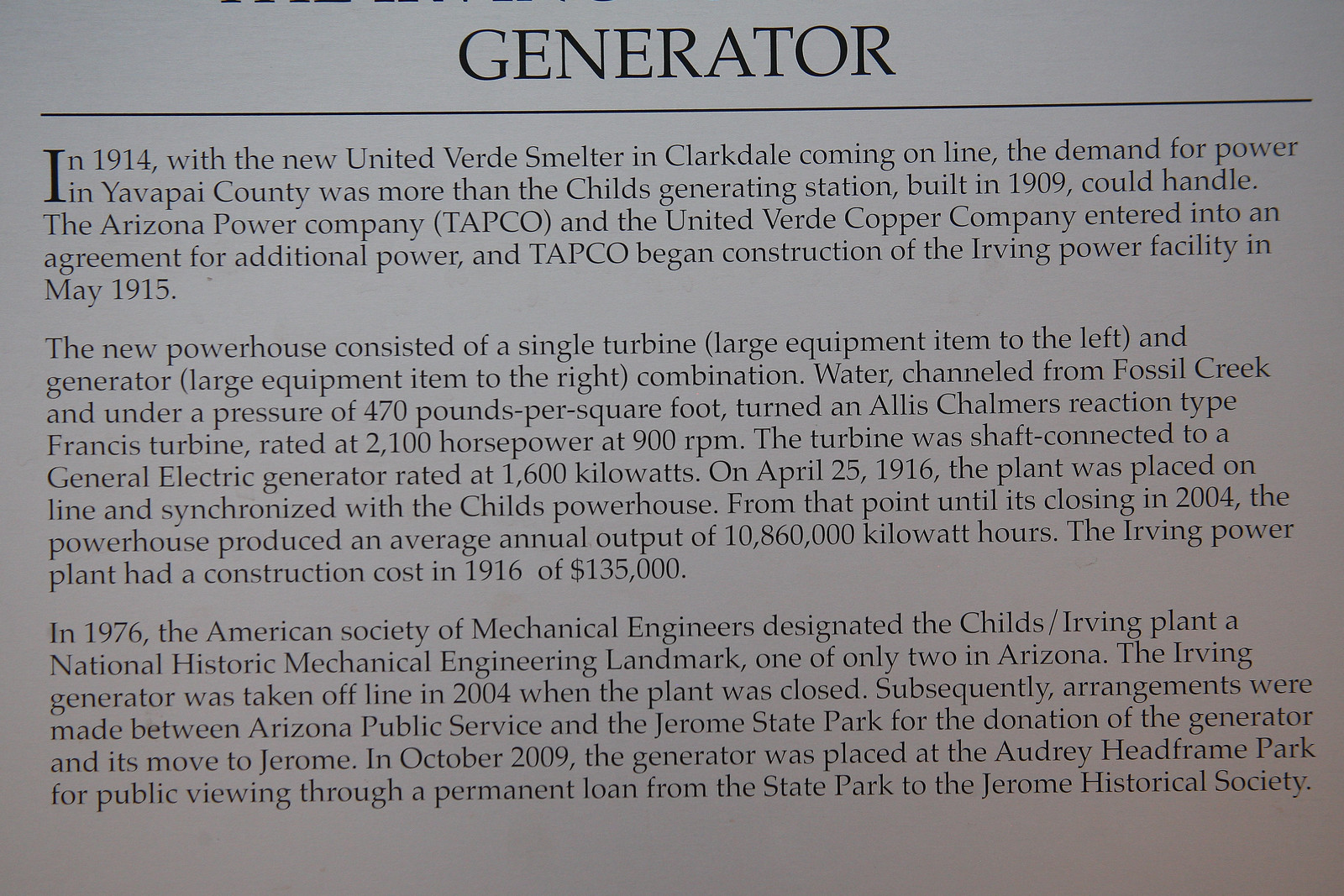The image depicts a detailed informative sign, likely found in a museum or historical exhibit, featuring an article titled "Generator." The content is presented in black text on a white background, divided into three paragraphs. The article describes the history of energy development in Yavapai County, Arizona. It explains how, in 1914, the new United Verde smelter in Clarkdale increased the demand for power beyond the capacity of the child's generating station, built in 1909. To meet this demand, the Arizona Power Company (TAPCO) and the United Verde Copper Company agreed to construct the Irving Power Facility. Construction began in May 1915 and included a single turbine and generator utilizing water from Fossil Creek. This water, channeled and pressurized to 470 pounds per square inch, powered an Alice Chalmers reaction type Francis turbine rated at 2100 horsepower and operating at 900 RPM. This sign conveys the historical significance of the turbine and its role in power generation in early 20th-century Arizona.